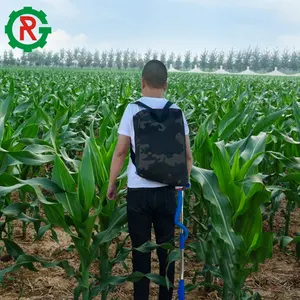In this square photograph, a boy stands facing away from the viewer in the middle of a vast cornfield. He is dressed in dark wash denim jeans, a white t-shirt, and carries a camouflage backpack. His short dark hair is closely cropped, revealing a shaved head. The corn plants rise to about his waist, filling the foreground and stretching towards the horizon. He is holding a metal rod with blue tubing in his right hand, possibly a farming tool or an injector for fertilizer or herbicide. The field is punctuated with rows of green stalks, eventually giving way to a dirt path at the very front of the image. In the distance, a row of pine trees lines the horizon under a blue sky dotted with clouds. Just before the trees, an industrial irrigation sprayer is visible, emitting a fan-like spray pattern from multiple heads. In the top left corner of the photograph, there is a green, textured logo resembling a wheel or partial circle with a red, stylized letter "R" or possibly "G" embedded inside.